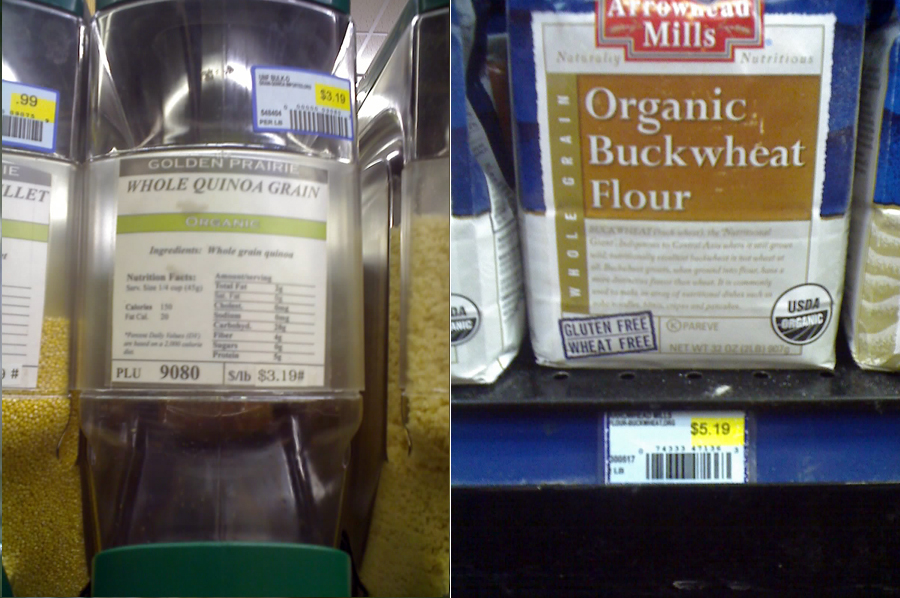The image displays two side-by-side photographs of products on market shelves. The first photograph features a large container of Golden Prairie Organic Ingredients Whole Grain Quinoa, with a label showcasing a yellow sticker pricing it at $3.19 per pound. The label at the top includes the PLU number 9080, and the quinoa grains are visible through the container. Adjacent to this is another container, likely filled with millet, priced at $0.99, although the label is partially cut off. 

The second photograph depicts a package of Arrowhead Mills Organic Buckwheat Flour, which is gluten-free and wheat-free. The packaging is prominently marked with "USDA Organic" and the price tag reads $5.19. The package's background is brown with black, white, and red text proclaiming its natural nutrition. The shelves under the products are black, further supporting the organized display.